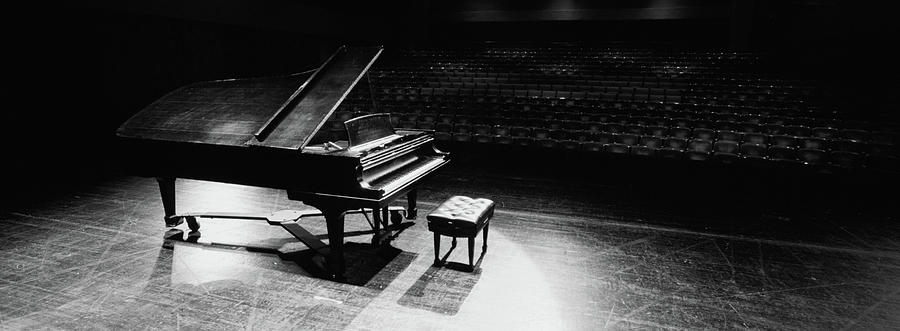This black-and-white photograph captures a grand piano positioned center stage in an empty theater. The piano is open, exposing its inner mechanics, and there's a sleek, low leather stool positioned in front of the keys. The stage itself, made of hardwood, appears well-used, evident from the numerous scratches and grooves across its surface. A single spotlight illuminates the piano and the stool, casting soft shadows and highlighting the details of the scene. In the background, rows upon rows of empty seats stretch out into a dimly lit, cavernous auditorium, emphasizing the absence of an audience and creating a sense of stillness and solitude. The theater's darker, overhead lights add to the moody ambiance, making the empty seats and the solitary piano the focal points of this evocative image.